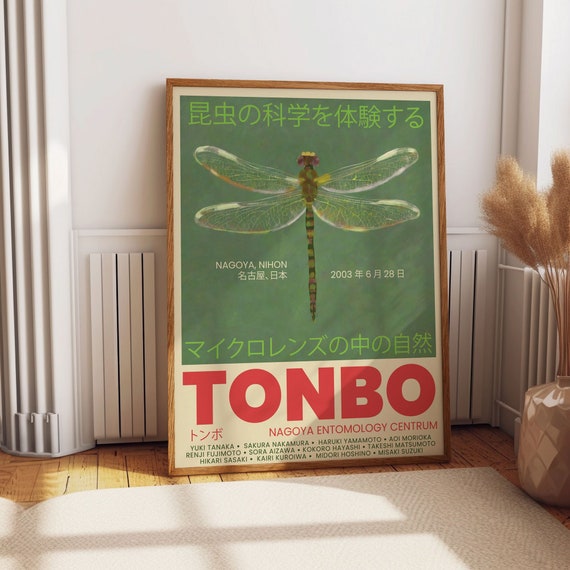The image is a large rectangular poster, propped against the wall in a room with a boho-chic ambiance enhanced by neutral tones and natural lighting. The white walls, adorned with white wood panels at the base, are complemented by a white rug on the brown hardwood floor. A small plant in a gray or tan pot adds a touch of nature to the setting.

The poster itself is striking, with a wooden frame and a vibrant design showcasing a prominent dragonfly, green and brown in color, with yellow and black accents on its face and wings. The dragonfly is set against a green background, accompanied by Japanese characters and some English text in red at the bottom that reads "Tanbo." Additional details include the location "Nagoya, Nihon," a date "6-28-2003," and the mention of the "Nagoya Entomology Centrium," suggesting it may be an advertisement or an old-school movie poster linked to an entomology event or research presentation. The clarity and detail of the image make it visually engaging, standing out vividly in the well-lit room.